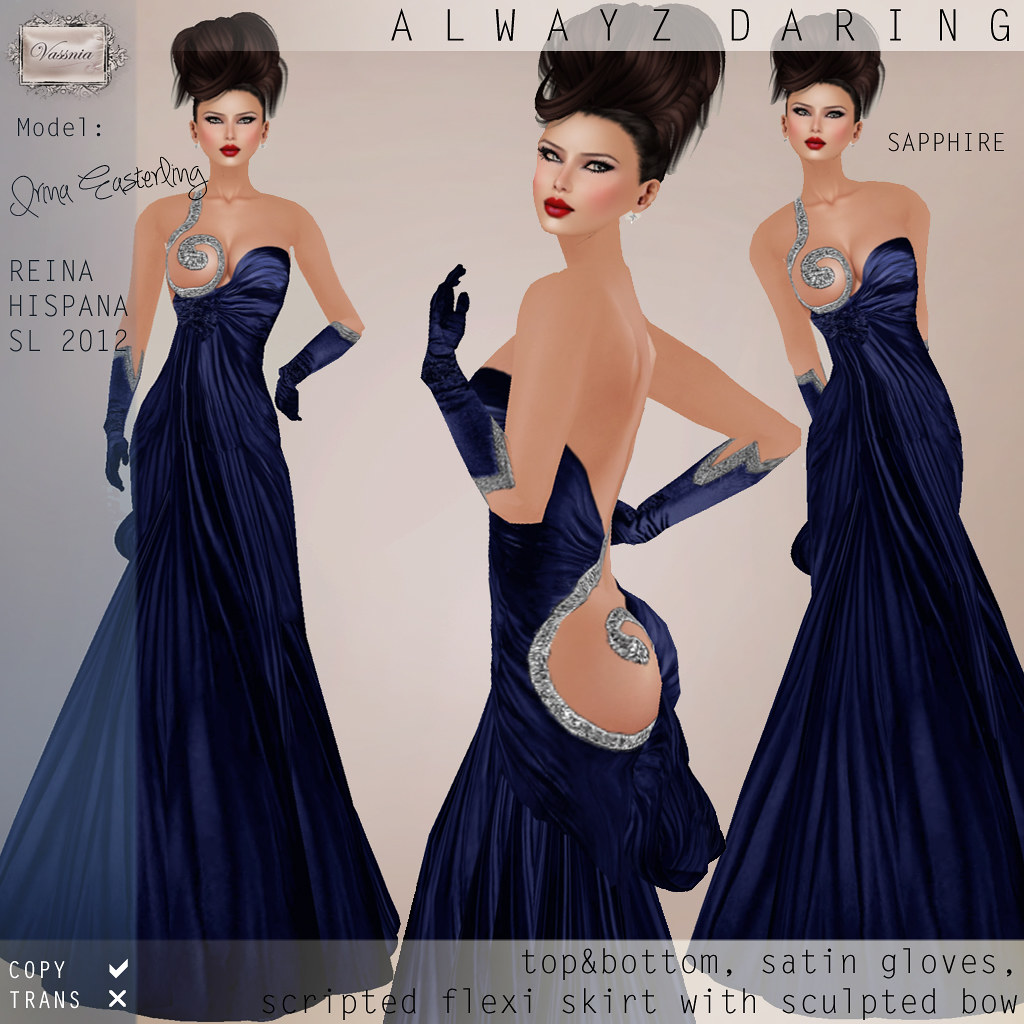This image features a detailed concept art drawing of a model named Irma Easterling, depicted wearing an elegant blue dress with unique design elements. The composition showcases her three times, emphasizing different angles and aspects of the attire. The dress is notable for its daring design, featuring a sparkly silver swirl that artistically covers her right breast, and another swirl pattern on her left lower cheek. The gown, which is deeply cut in the back, is complemented by matching blue satin gloves ideal for formal occasions such as a wedding or opera. Irma has high, styled black hair and wears striking red lipstick, accentuating her model-esque appearance. The artistic portrayal is described with several captions in the image: "Always Daring" is inscribed at the top right, alongside the word "Sapphire." At the bottom right, detailed in black text, are the features of her outfit: "Top and Bottom, Satin Gloves, Scripted Flexi Skirt with Sculpted Bow." The bottom left includes a note in white text, "Copy ✓" and "Trans X." The top left identifies the model's name in cursive, followed by "Reyna Hispania SL 2012."